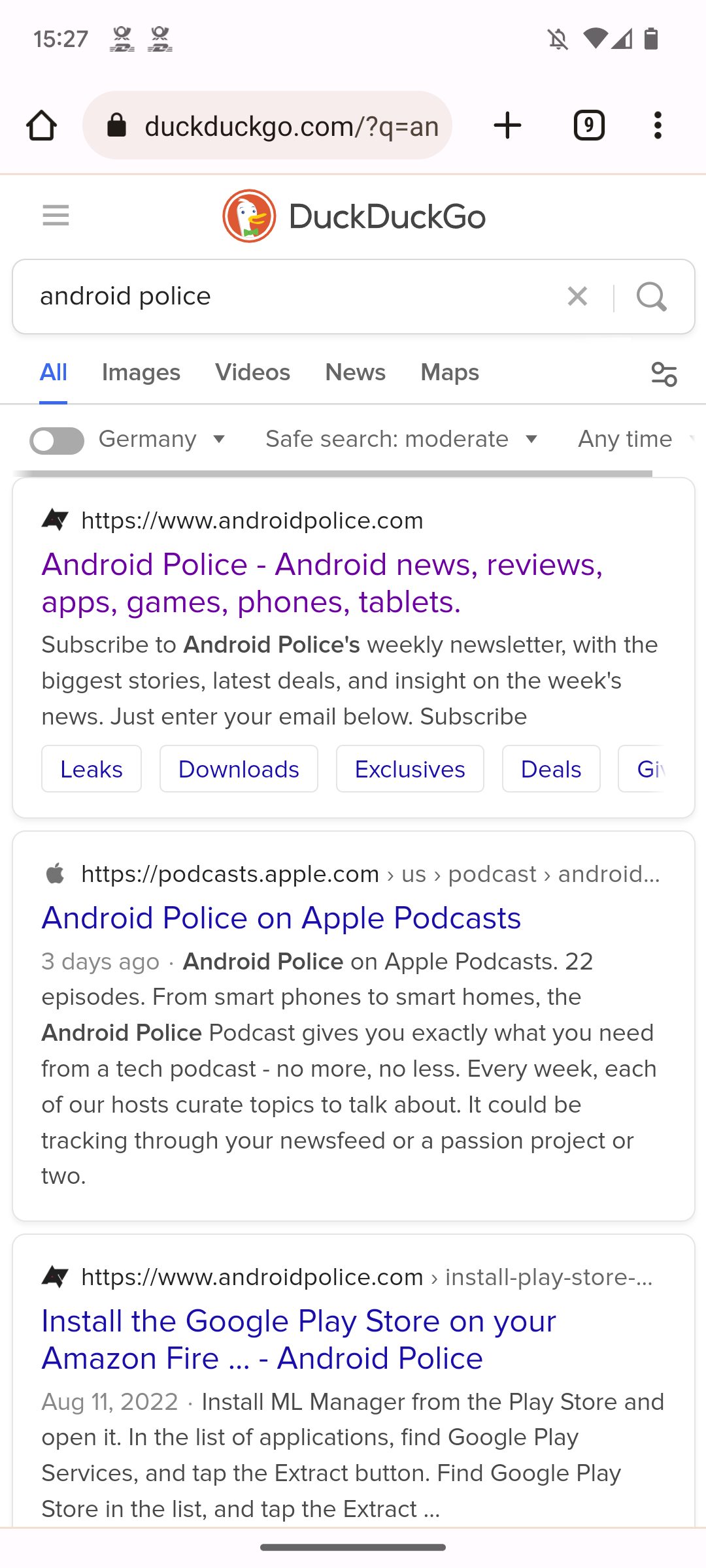The image depicts a search results page for the query "Android Police" on the Tuk Tuk Go browser. The time is 3:27 PM, displayed at the top left corner of the screen. On the right side, the status bar features icons for silent mode, WiFi signal strength, network signal strength, and battery level.

The first search result is a link to "androidpolice.com," with the description "Android Police: Android news, reviews, apps, games, phones, tablets." This link appears in purple, indicating it has been previously visited, contrast to unvisited links that would typically appear in blue.